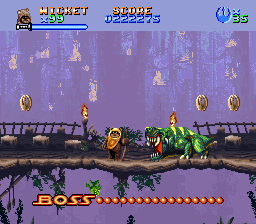This image appears to be a screenshot from an older, pixelated video game, likely from the 80s or early 90s, reminiscent of those found on platforms like Nintendo or Sega. The scene suggests a Star Wars-themed game, potentially featuring an Ewok named Wicket as the playable character. In the top-left corner, the caption "Wicket" is displayed in a yellow and orange gradient, accompanied by an icon of Wicket and a statistic reading "x99" in neon green. To the right of the screen, a trident icon is marked "x35".

The main action takes place on a wooden bridge that is adorned with hanging vines and tree stumps. The bridge itself features wood railings and a centrally located torch. The background is a forest scene with faded trees, and the overall screen hue appears to be purple or blue. Suspended in the air above the bridge are three coins—one on the left and two on the right.

The centerpiece of the scene is Wicket, recognizable by his orange hood, standing on the bridge facing a green, tiger-like predator. At the bottom of the screen, the word "Boss" is highlighted in yellow, followed by several little flame icons. Across the top middle of the screen, the score is displayed as "0222275." This screenshot embodies the classic retro gaming aesthetic, complete with pixelated graphics and a nostalgic atmosphere.